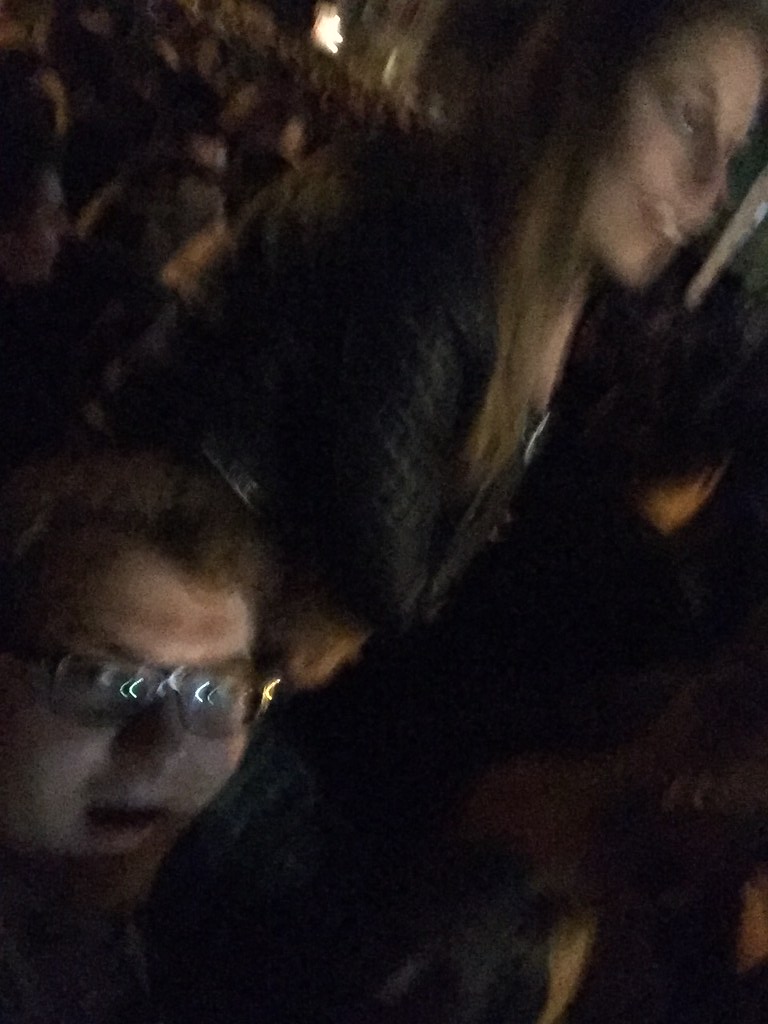The image depicts an outdoor nighttime gathering, featuring a dense crowd of heads. In the foreground, there's a young man situated in the lower left corner. He has curly brown hair, glasses with reflections of light—showing a mix of white and greenish hues—and is possibly smiling with his mouth slightly open. Beside and slightly above him to the right, there is a woman with shoulder-length hair, which might be either blonde or light brown, wearing a black leather jacket. She appears to be smiling as well. The scene is dimly lit, with the faces of the two individuals being the most prominent, illuminated parts of the image, while the rest of the crowd blends into the dark background. The camera angle is slightly tilted, adding to the dynamic, somewhat blurry nature of the photo.